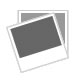The photograph showcases a pair of medieval armor gauntlets with intricately designed, shiny metal that covers each finger, wrist, and palm. The gauntlets feature pointed knuckles and spiked metal points at the joints, emphasizing their detailed craftsmanship. The thumb design appears mechanical, with clip-like ends, which further adds to the impression of sophistication in their construction. The textured ridges running along the hand and wrist sections resemble the look of tin cans and likely serve both decorative and practical purposes. These gleaming gauntlets are laid out on an olive green backdrop, which is torn and marred by brown and black spots, scratches, and scrapes, enhancing the contrast between the weathered surface and the pristine condition of the armor. This juxtaposition suggests the gauntlets might be newly made or recently refurbished, standing out vividly against the well-used background.